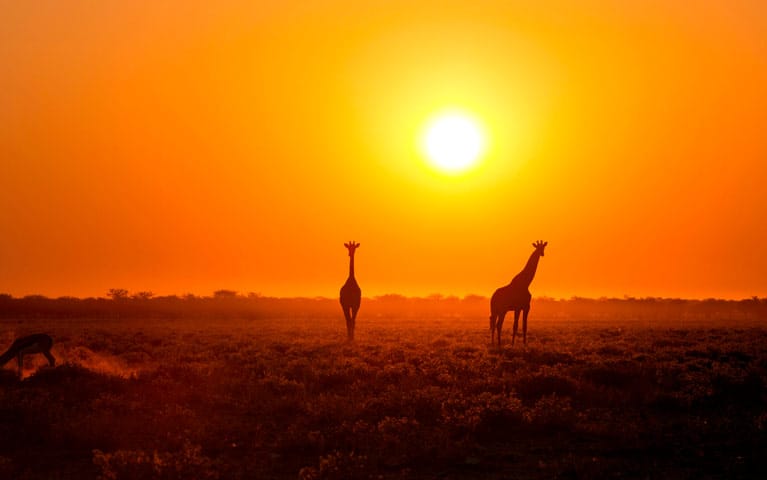This photograph, captured in the late afternoon on an African safari, presents a compelling landscape layout showcasing the vibrant hues of a setting sun. The top half of the image is dominated by a gradient sky, transitioning from a white-centered sun through shades of yellow to deep orange at the edges. The sun sits precisely in the center, radiating warmth and color over the serene scene. Below, the flat, dry grassland extends across the image, shadowed in near darkness but delicately lit by the ambient glow. 

In the foreground, two giraffes are prominently silhouetted, creating iconic and majestic shapes against the colorful sky. The giraffe on the left is seen from behind, showcasing a tall neck and body outline, while the one on the right stands in profile, its full form captured in a side glance toward the camera. Some distant trees mark the horizon, blending subtly into the transition between land and sky. Additionally, a smaller shape with a long neck suggests the presence of a baby giraffe beside them, adding a tender element to the scene.

Overall, the photograph portrays the tranquil beauty and natural splendor of the African savanna, where the silvery silhouettes of giraffes enhance the enchanting palette of a fading day.